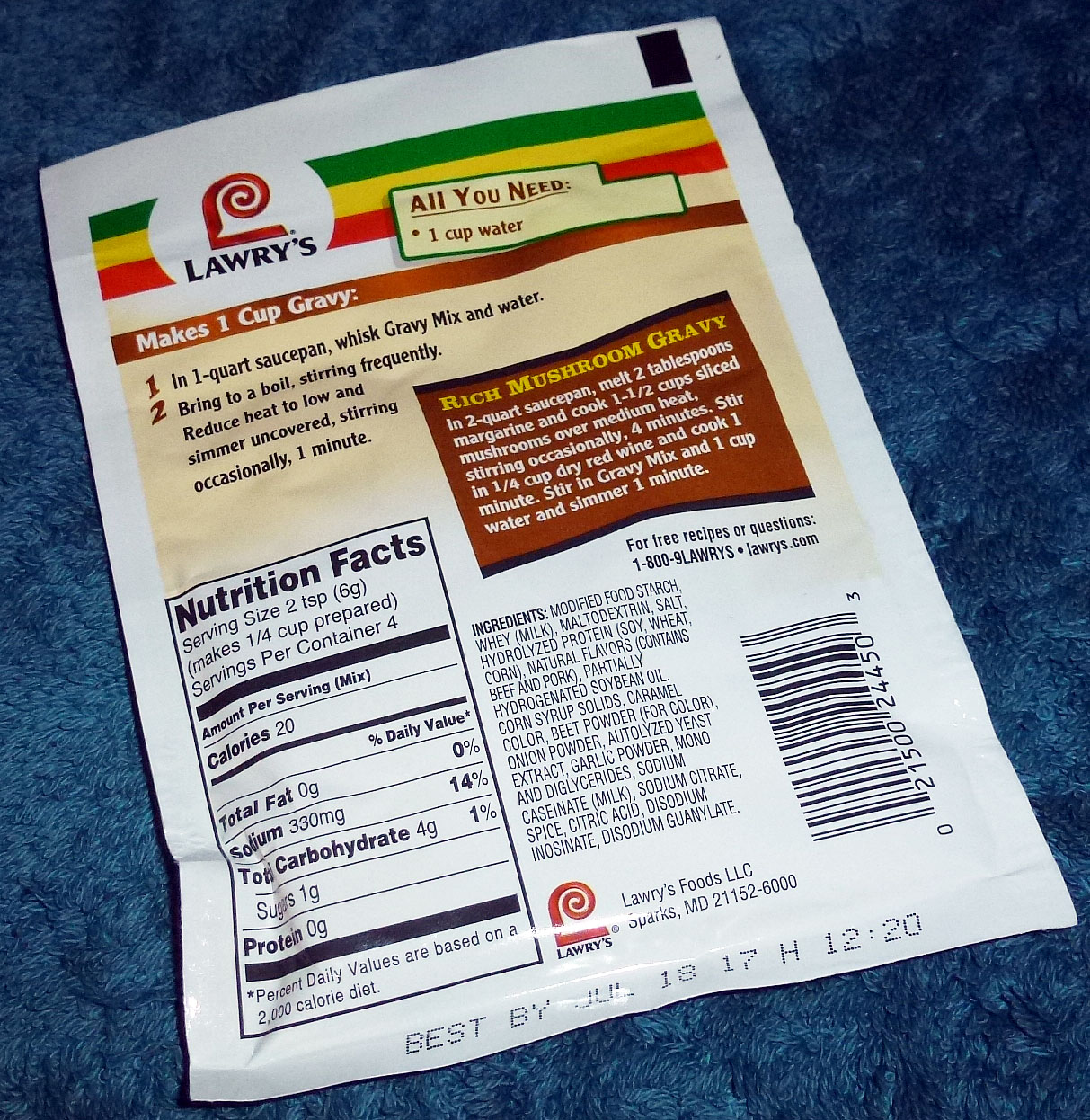The image depicts the backside of a seasoning packet from Lori's. The detailed instructions on the packet indicate that this seasoning mix produces one cup of gravy. The preparation steps are clearly outlined in two parts: 

1. In a one-quart saucepan, whisk together the gravy mix and water.
2. Bring the mixture to a boil while stirring frequently, then reduce the heat to low and simmer uncovered for one minute, stirring occasionally.

Additionally, the packet includes nutritional information, a recipe for rich mushroom gravy, and a comprehensive ingredient list. A barcode is positioned on the right corner of the packet, along with a "best by" date of July 18, 2017, accompanied by a letter and a time stamp. The packet itself is placed on a blue, fluffy surface, enhancing the visual appeal of the image.